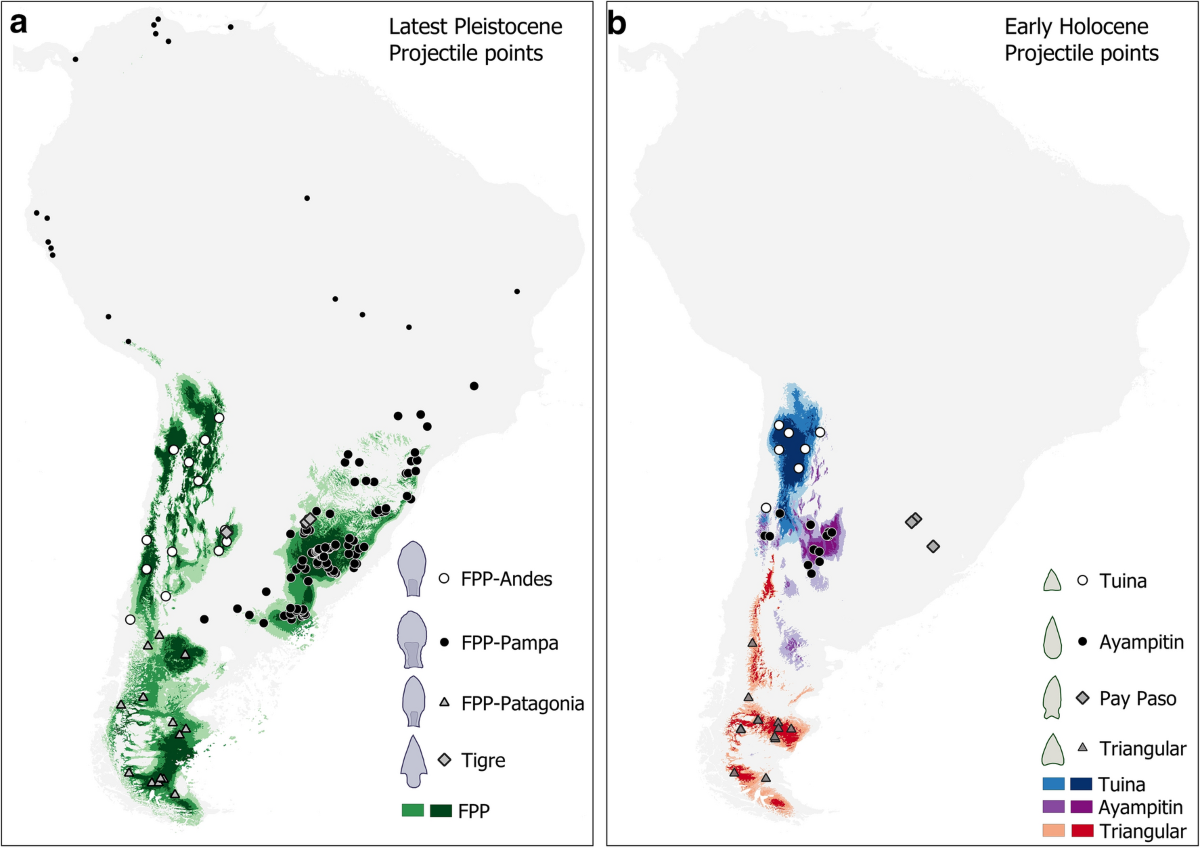The image features two maps of South America, labeled A (on the left) and B (on the right), each bordered in black on a white background. Map A, marked with a lowercase 'a' in the top left corner, displays the continent titled "Latest Pleistocene Projectile Points" in black lettering at the top right. Its legend at the bottom right explains the use of circles, triangles, and diamonds that likely represent different types of animal life. The map is colored in various shades of green—light, medium, and dark—concentrated towards the bottom of South America.

On the right, Map B, identified by a lowercase 'b' in the top left corner, is almost identical in layout but focuses on a different time period, titled "Early Holocene Projectile Points" at the top right. This map utilizes a spectrum of colors including blues, reds, purples, and oranges, differentiated into light, medium, and dark shades to illustrate changes over time. Like Map A, Map B also employs circles, triangles, and diamonds to represent various species across the continent. Each map includes a legend at the bottom right for reference.